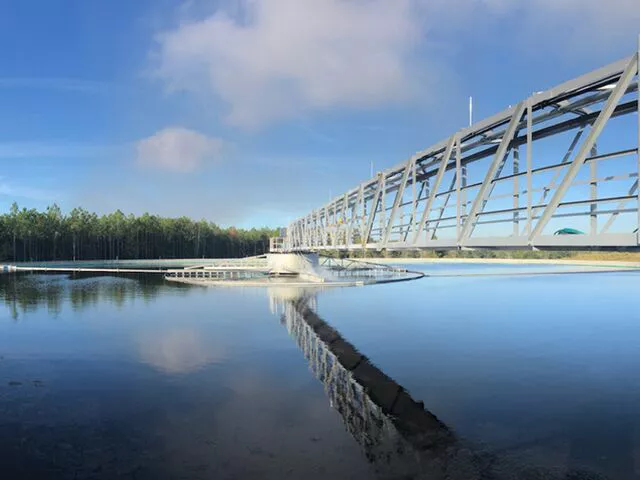This photograph captures a serene, sunlit scene featuring a slender, gray pedestrian bridge, constructed with angled protective beams forming a zigzag pattern on both sides. The bridge stretches from the right side of the image towards the center, culminating in a circular structure of similar material, likely a loading ramp. The bridge and its intricate design are mirrored in the calm, blue water below, which also reflects the slightly gray, wispy clouds from the cyan and light blue sky above. Flanking the left side of the image is a lush, expansive tree line, its verdant greenery towering towards the sky and also mirrored on the water's surface. A notable cyan piece of material is visible on the right side of the bridge, adding a pop of color to the metallic scenery. The backdrop features what appears to be a secluded island of trees, enhancing the overall tranquility of the idyllic setting.